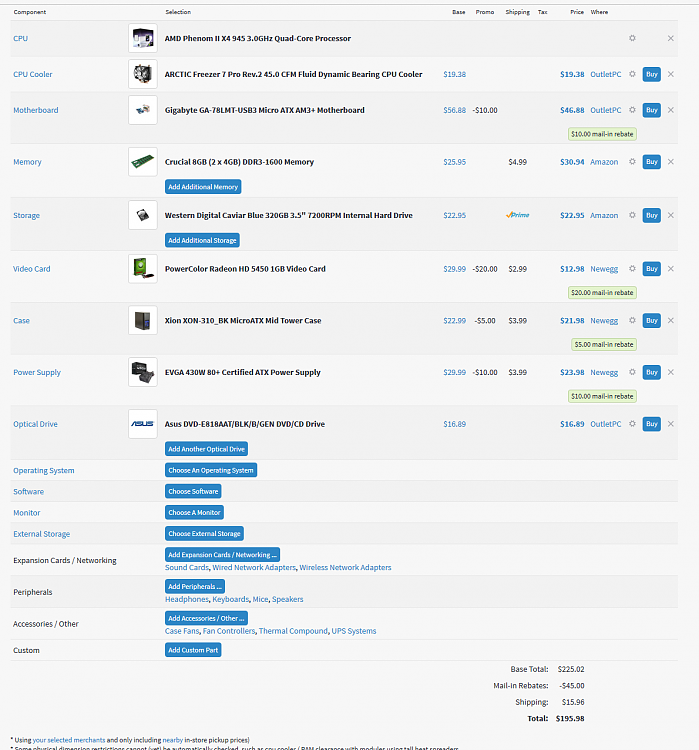This image depicts a comprehensive components list for building a custom computer system. Each component is meticulously detailed to provide an overview of the hardware necessary for assembling a high-performance unit. The specific components and their respective specifications are as follows:

1. **Processor:** AMD Phenom II X4 945 Quad-Core, operating at 3 GHz, providing robust processing power.
2. **CPU Cooler:** Arctic Freezer 7 Pro Rev. 2, featuring CFM fluid dynamic bearings for efficient heat dissipation.
3. **Motherboard:** Gigabyte 780LMT with USB 3.0 and micro HDMI 3.0 capabilities, ensuring modern connectivity and expansion options.
4. **Memory:** Virtual HDB 2 x 4GB, DDR 3600, offering rapid data access speeds to enhance overall system performance.
5. **Storage:** Western Digital Blue, 328GB, 3.5" hard drive, spinning at 7200 RPM for reliable data storage and retrieval.
6. **Video Card:** PowerColor Radeon HD 5450, providing capable graphics rendering for everyday tasks and light gaming.
7. **Case:** AC on XLM 310, a micro ATX mid-tower case, offering a balance of compact form and interior space for components.
8. **Power Supply:** EVGA 430W, 80 Plus certified, ensuring efficient power delivery to all system components.
9. **Optical Drive:** Not specified, but indicative of considerations for potential inclusion depending on user needs.
10. **Operating System:** Not specified, but integral to the build, ensuring the necessary environment for software operations.
11. **Software:** Not specified, potentially covering a range of applications essential for varied use cases.
12. **Monitor:** Not specified, but essential for visual output of the system.
13. **Peripherals:** Not specified, but could include essentials like a keyboard, mouse, and other input devices.
14. **Networking:** Not specified, but typically includes options for wired or wireless internet connectivity.
15. **Expansion Cards:** Not specified, leaving room for future enhancements to system capabilities.
16. **External Storage:** Not specified, considering additional data storage expansion beyond internal capacities.

The list is indicative of a methodical selection of components to assemble a functional and efficient computing system tailored to specific performance and usability needs.